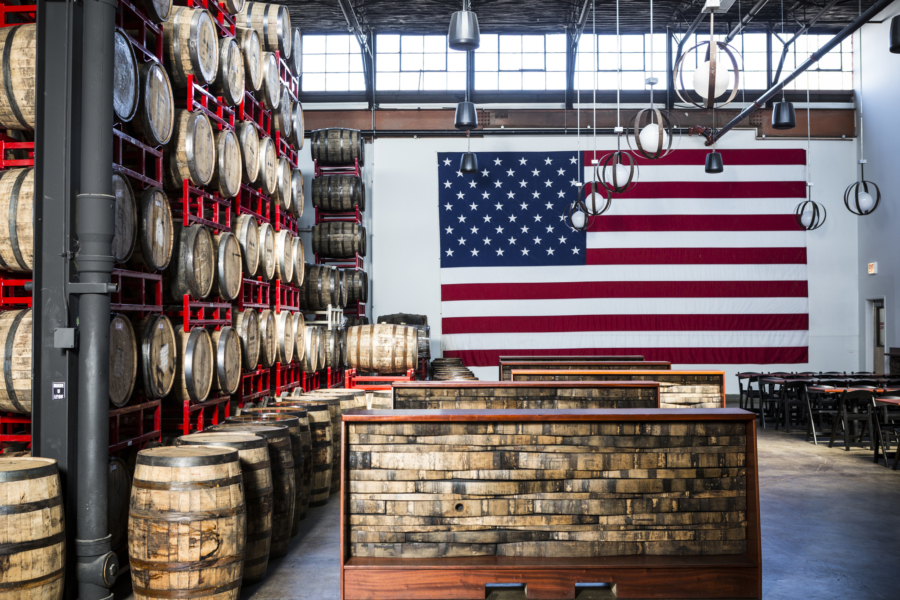The image depicts the interior of a large industrial warehouse, possibly a winery or whiskey distillery, with a distinctly patriotic atmosphere highlighted by a huge American flag adorning a white wall in the background. The spacious room features numerous wooden barrels, all with metal strappings, some stacked on the concrete floor and others lined up on red metal racks, indicating where the aging process of the substance—likely liquor or beer—takes place. The warehouse is illuminated by industrial-style, bulbous lights hanging from the ceiling, enhancing the utilitarian look of the space. On the right-hand side, tables and chairs, possibly used for tastings or as a lunch area, are neatly arranged, adding a functional touch to the room. In front of the barrels and the American flag, various cases and boxes are scattered, possibly holding materials or unfinished barrels, contributing to the industrial yet organized ambiance of the facility.